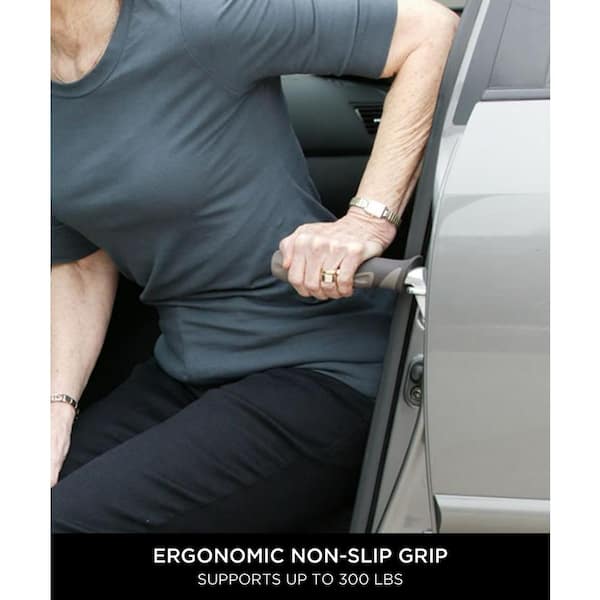This image showcases an elderly Caucasian woman in a silver van, using an ergonomic, non-slip grip tool designed to aid in exiting vehicles, which supports up to 300 pounds. She is wearing a gray t-shirt with elbow-length sleeves and black pants. Her left hand, adorned with a silver wristwatch and a ring on her ring finger, is gripping the metal handle attached to the car door. This tool, resembling a bicycle handle, hooks onto the door latch to provide additional support for individuals, particularly useful for taller vehicles like vans and pickup trucks. The woman’s pale, slightly wrinkled arms and the detailed description of the assistive device emphasize its utility in helping older adults safely get in and out of their cars.